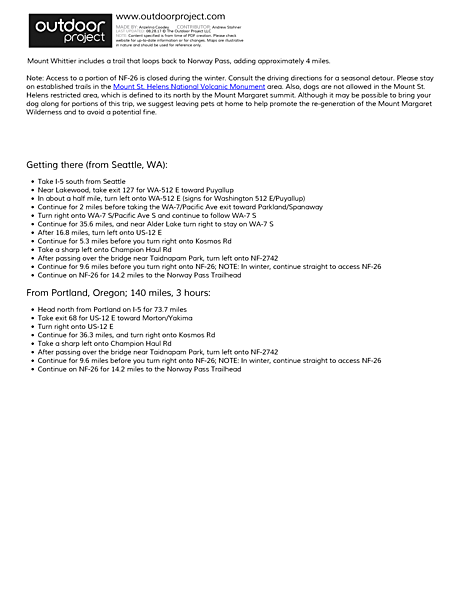The image features a white background with the text "Outdoor Project" displayed in white letters on a black rectangle, alongside the website "www.outdoorproject.com." There is a detailed description about Mount Witter, indicating that the trail includes a loop back to Norway Pass, adding approximately four miles. The image contains a blue hyperlink to information about the Mount St. Helens National Volcanic Monument. Directions for getting there from Seattle, Washington, include:

- Head south from Seattle near Lakewood.
- Take exit 127 for Washington and then S12E heading east.
- Note: There is a potentially misspelled or unclear place name, possibly referring to Puyallup (p-u-y-a-l-l-u-p).

Additionally, directions from Portland, Oregon are mentioned, noting a distance of 140 miles and an approximate travel time of three hours. There is also a bullet-point list providing further navigational details.